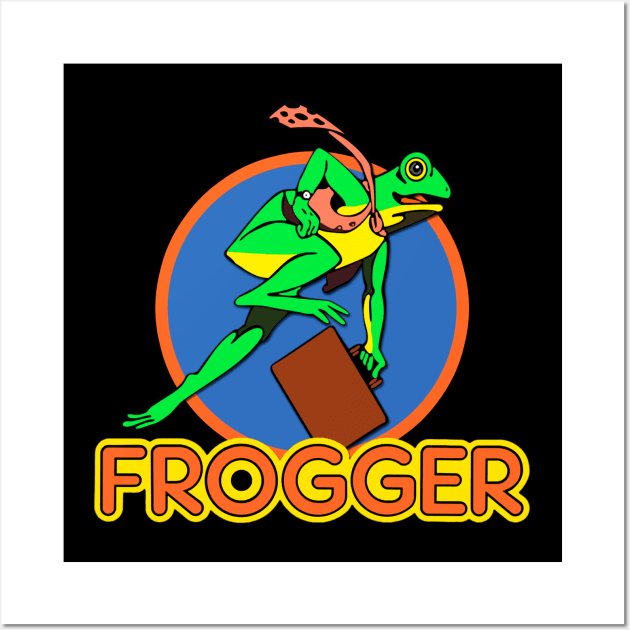This is a detailed poster for the game "Frogger." The background is a black square, making the vibrant colors of the design stand out strikingly. At the center of the poster, there's a blue circle with a burnt orange outline. Inside this circle, a green frog with a yellow belly is depicted running frantically, as if he's about to miss the bus. The frog is dressed in a distinctive salmon-colored polka dot tie and a wristwatch on his right wrist. He clutches a brown briefcase in his left hand. Below the circle, the word "Frogger" is prominently displayed in big, retro-style bubble letters, primarily salmon in color with a yellow outline. The 'O' in "Frogger" features a black center, adding to the arcade-style aesthetic. Overall, the vibrant colors and nostalgic design elements make this poster a striking advertisement for the "Frogger" game.